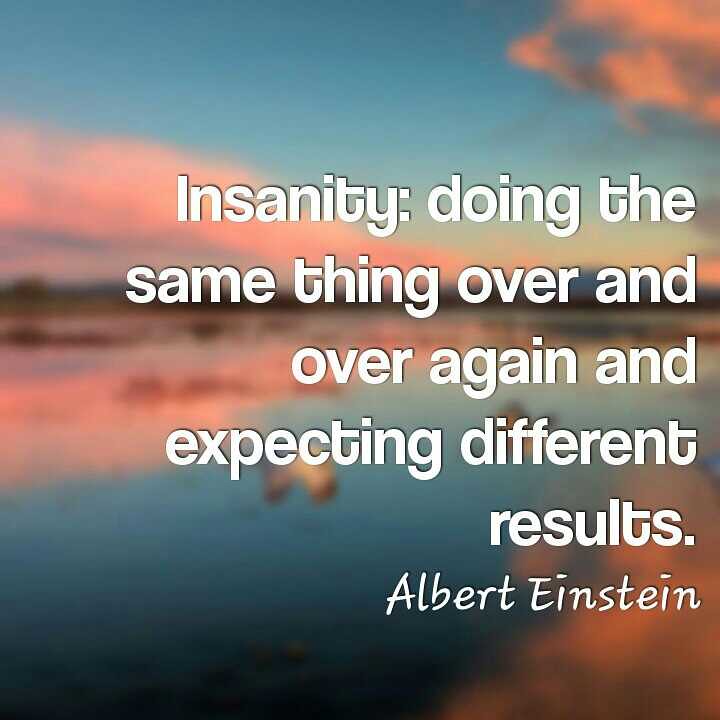This image is a motivational quote commonly seen online, featuring an attributed quote by Albert Einstein: "Insanity: doing the same thing over and over again and expecting different results." The quote is displayed in blocky white letters with "Albert Einstein" in a cursive font. The background is a blurry photograph of a sunset or sunrise over a beach, characterized by reddish and orangish-pink clouds reflected in the water below. Despite the lack of resolution in the background, the text remains the primary focus, filling the image from top to bottom, slightly indented on the right-hand side. The overall composition and blurred scenery add a serene yet contemplative quality to the inspirational message.